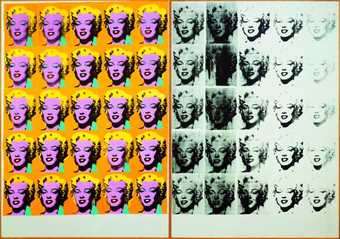This close-up photo showcases Andy Warhol's "Marilyn Diptych," featuring two vertically-aligned grids of simplified, retro face portraits of Marilyn Monroe. Each grid is composed of 25 images arranged in five rows and five columns. On the left side, the images are colorful with Marilyn's face in a pinkish skin tone, blonde hair, pink lips, light cyan-green eye makeup, and an orange background, along with a light blue earring in each portrait. On the right side, the images are in grayscale, gradually becoming more faded and distorted towards the right, losing detail and clarity. Despite the decaying effect on the right-hand side, both grids present almost identical images of Marilyn Monroe, emphasizing both the vibrant details and the stark, deteriorating contrast.